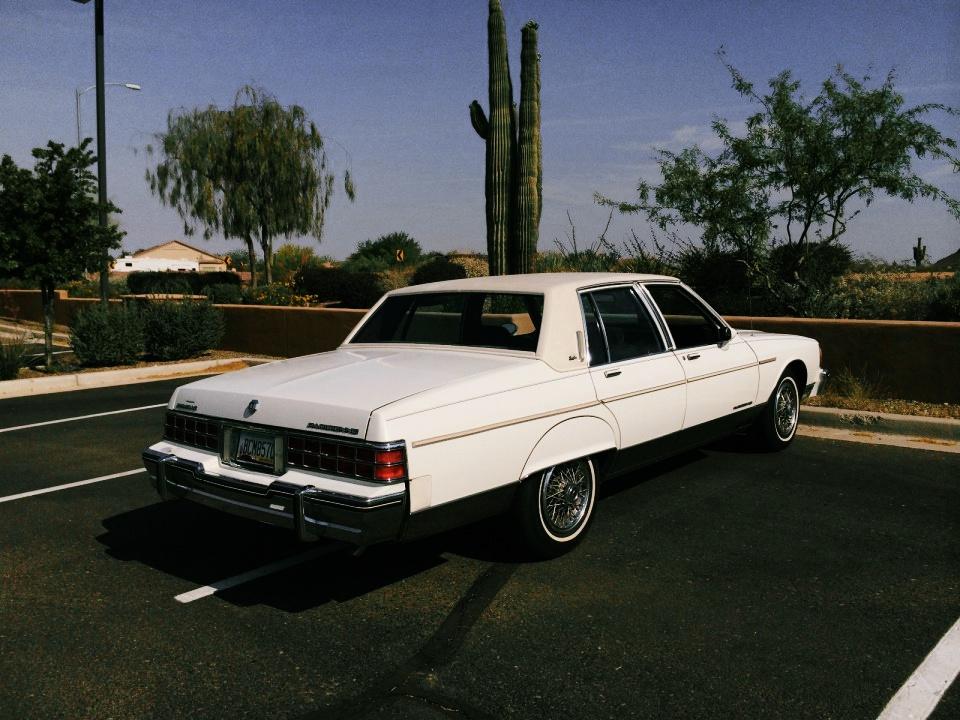A classic, older model four-door white sedan, possibly a Buick or a Pontiac, is parked in the center of a blacktop parking lot, straddling a white painted line, indicating it is taking up two spaces. The car features a gold pinstripe running from the front wheel to the back, whitewall tires, and a long, squared-off trunk. The rear license plate is visible, though unreadable. The top of the car appears cream-colored, contrasting with its otherwise white body, and the tail lights are red. Its position shows the car facing towards the upper right corner of the image at a 45-degree angle, emphasizing the rear and right side.

In the background, directly in front of the car and slightly to the left, stands a large green cactus, framed by a bright, dark-blue sky with wispy clouds. To the left of the image, a telephone pole and a triangle-shaped building are visible in the distance, while sparse, dried green shrubbery and a few dark green, scraggly trees populate the surrounding area, indicating a likely desert setting. The car is parked facing a concrete retaining wall, situated about 10 to 20 feet away. The parking lot itself features three and a half visible white lines, with the half-line appearing on the right side of the shot.